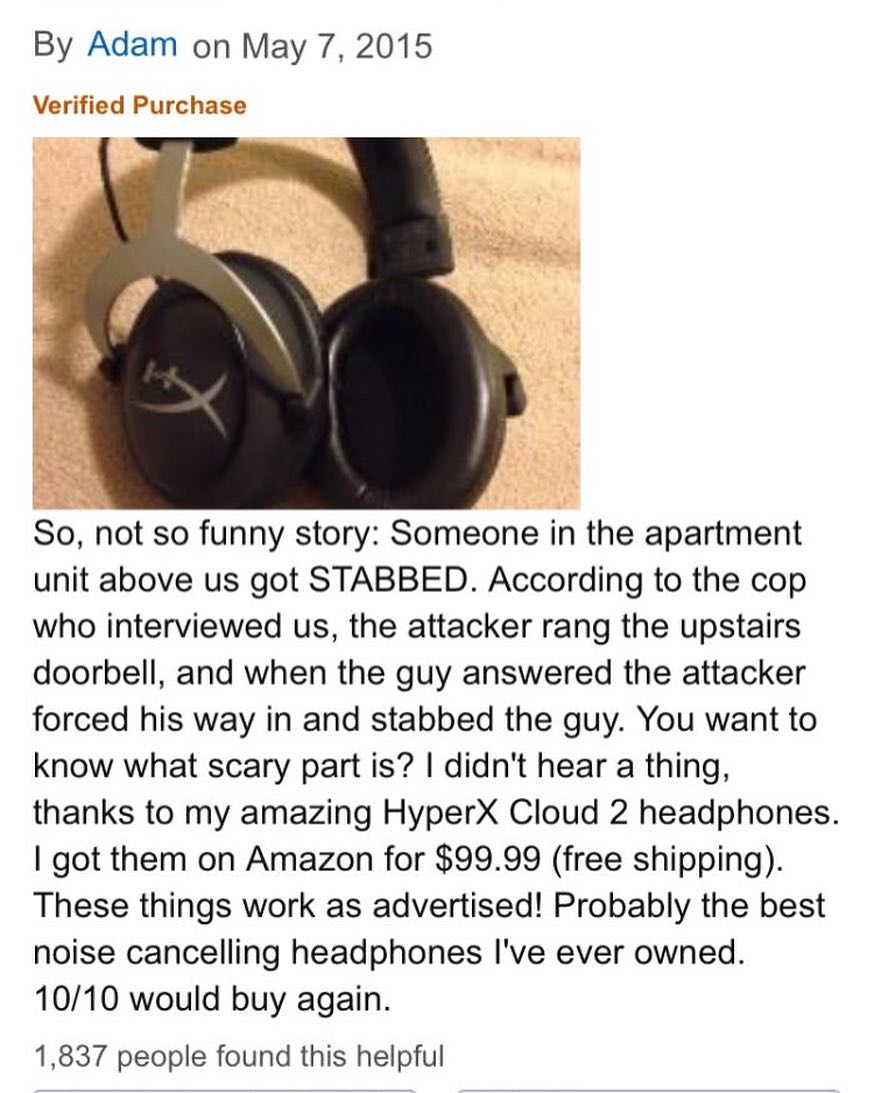This image is a screenshot of an Amazon review posted by Adam on May 7, 2015, marking a verified purchase. The photograph showcases the HyperX Cloud II headphones, predominantly black with silver accents, including an "H" with two white lines on one of the earpieces. The review recounts a disturbing yet striking testament to the headphones' effectiveness: Adam describes how, one night, someone in the apartment above him was stabbed when an attacker forced their way in after ringing the doorbell. Astonishingly, Adam did not hear a thing due to the outstanding noise-canceling capability of his HyperX Cloud II headphones, which he purchased for $99.99 with free shipping on Amazon. Adam praises these headphones as the best noise-canceling headphones he has ever owned, giving them a perfect score of 10 out of 10 and stating he would buy them again. The review ends noting that 1,837 people found this information helpful.